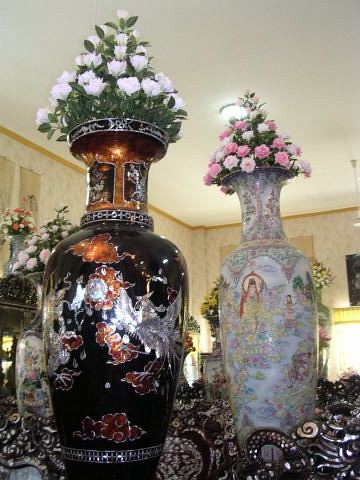In the image, there are two prominent flower pots set in a lavish, ornately decorated room. The pot on the left is black, adorned with intricate designs that include a bird motif and white flowers on top. This pot features detailed, old markings, possibly depicting religious figures or angels. To the right stands a light blue, almost powder blue, pot embellished with pastel colors including blues, yellows, and pinks. This pot showcases lavish decorations, possibly Asian holy figures, and has pink flowers on top. The room itself is grand with high ceilings and formal decor. The walls are covered in cream and gold patterned wallpaper, complemented by yellow molding and a plain cream ceiling. The floor is carpeted in black, and artificial indoor lighting illuminates the scene. In the background, additional vases with various designs and flower arrangements can be seen, adding to the room's opulent atmosphere. Scattered on the ground near the vases are metallic objects, resembling coins or dragon-themed decorations.